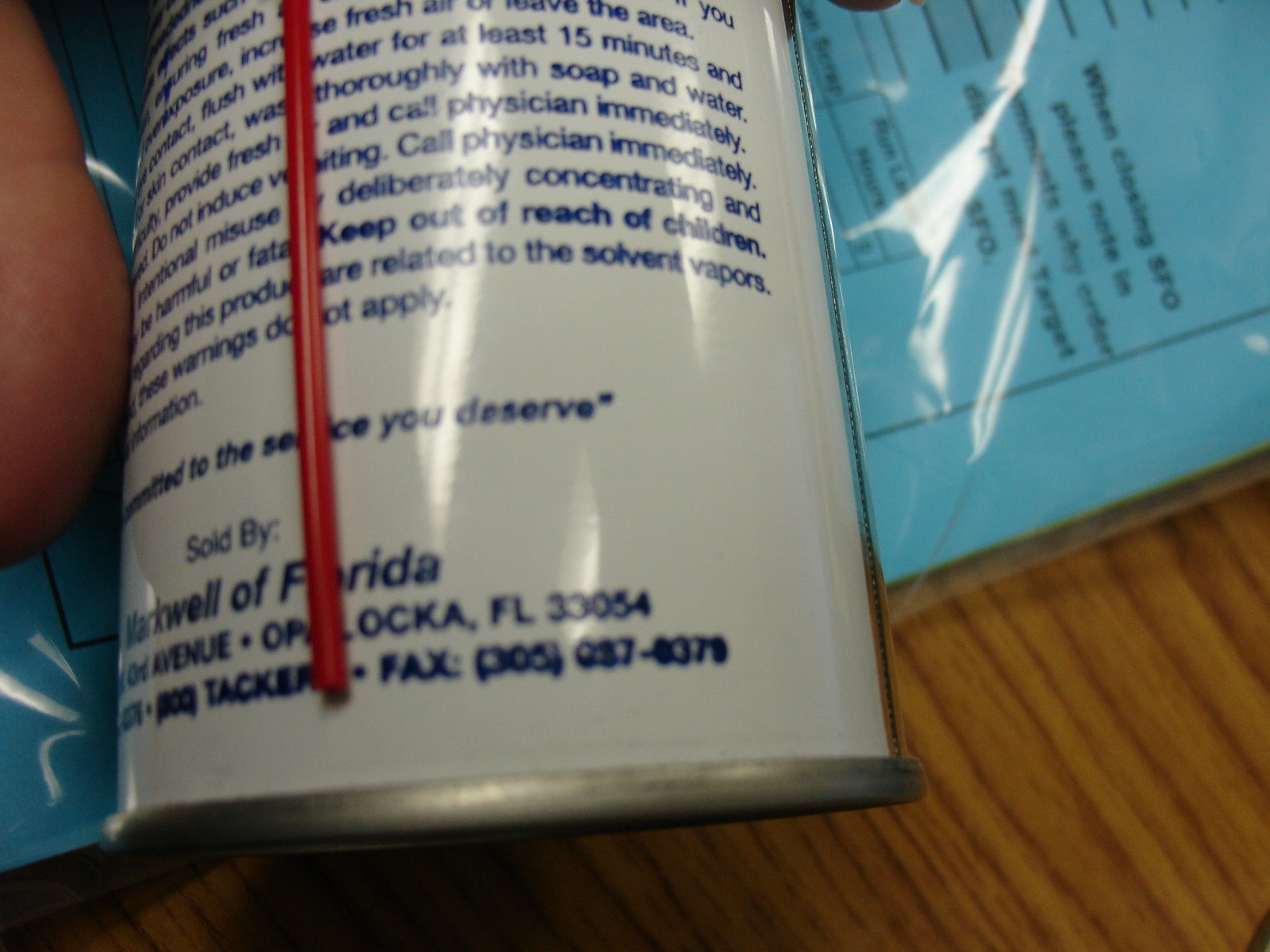The photograph depicts the back of an aerosol can situated on a brown table. The can features a silver bottom and a white label with blue text containing important safety instructions, including warnings about flushing with water for at least 15 minutes if the product makes contact with skin, thoroughly washing with soap and water, not inducing vomiting, calling a physician immediately, and keeping the product out of reach of children. A red straw, similar to those found on products like WD-40, is attached to the can for precise application. To the left of the image, a person's finger is visible near the top. In the upper right corner, extending downwards, is a clear plastic sheet protecting a blue piece of paper with black printed text and form-like boxes. The plastic cover reflects light at both its top and bottom portions. The word "Florida," a fax number, and additional information are also partially visible at the bottom of the can’s label.